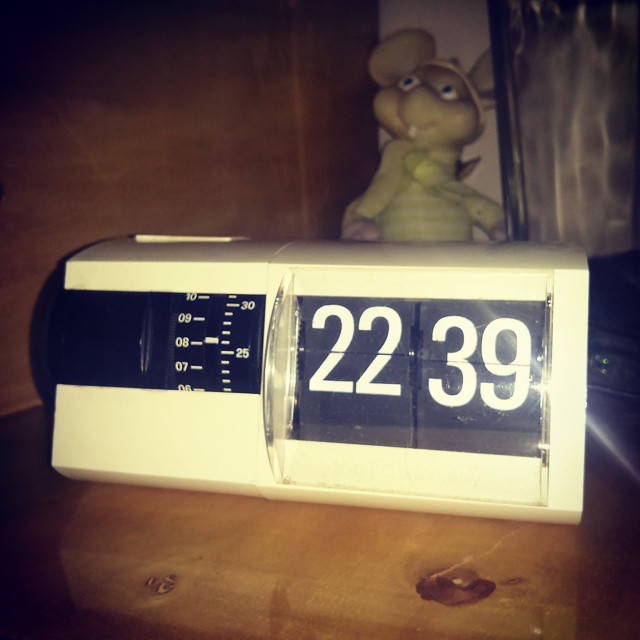In the foreground, the photograph features an old-school white analog clock displaying the time in military format as 22:39. The clock itself is placed on a varnished wooden table. To the left of the clock, there are black dials with white numbers, possibly for setting an alarm. The clock appears to have flip-style numbers and is housed behind a hard clear plastic covering. The table has a rich brown hue, complementing the white clock.

Behind the clock sits a light green figurine of a mouse with a mint green face, white and blue eyes, green ears, and a yellow-green scarf. The mouse has one prominent white tooth. To the right of this mouse figurine is an unidentified object in shades of black and white, while in the background to the top right, there's a wavy gray and white patterned fabric or curtain. The scene is illuminated with light reflecting off the clock face, and a brown storage area or closet is partially visible in the top left corner of the image.